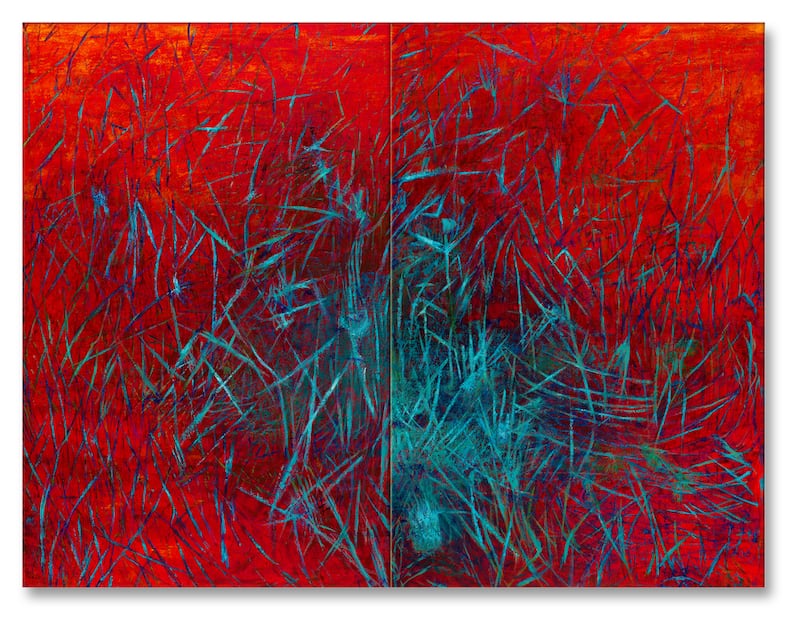This image showcases a captivating piece of abstract art that spans two pages. The vivid orange-red background serves as the canvas for intricate blue patterns. The blue strokes, resembling lines or scribbles, are denser toward the center of the composition, creating a concentrated focal point. These lines are meticulously drawn and vary in appearance, with some exhibiting shimmery brightness while others are more shadowed, adding depth and a sense of motion to the artwork. The distribution of blue becomes more dispersed and lighter as it extends outwards towards the edges of the pages.

The right page of the artwork is saturated with thick blue lines, particularly along the left side, gradually thinning as they spread out. In contrast, the left page features a lighter application of blue, allowing the individual stripes to be more discernible and also becoming lighter as they reach the edge. There is a slight difference in the background tones, with the right half incorporating more yellow highlights compared to the left.

The overall arrangement of the blue lines evokes imagery that can be interpreted in various ways—some might see hands reaching out, scratches made by claws, or even stick figures. This rich, textured painting effectively blends the vibrant background with detailed blue strokes to create a dynamic and visually engaging piece.